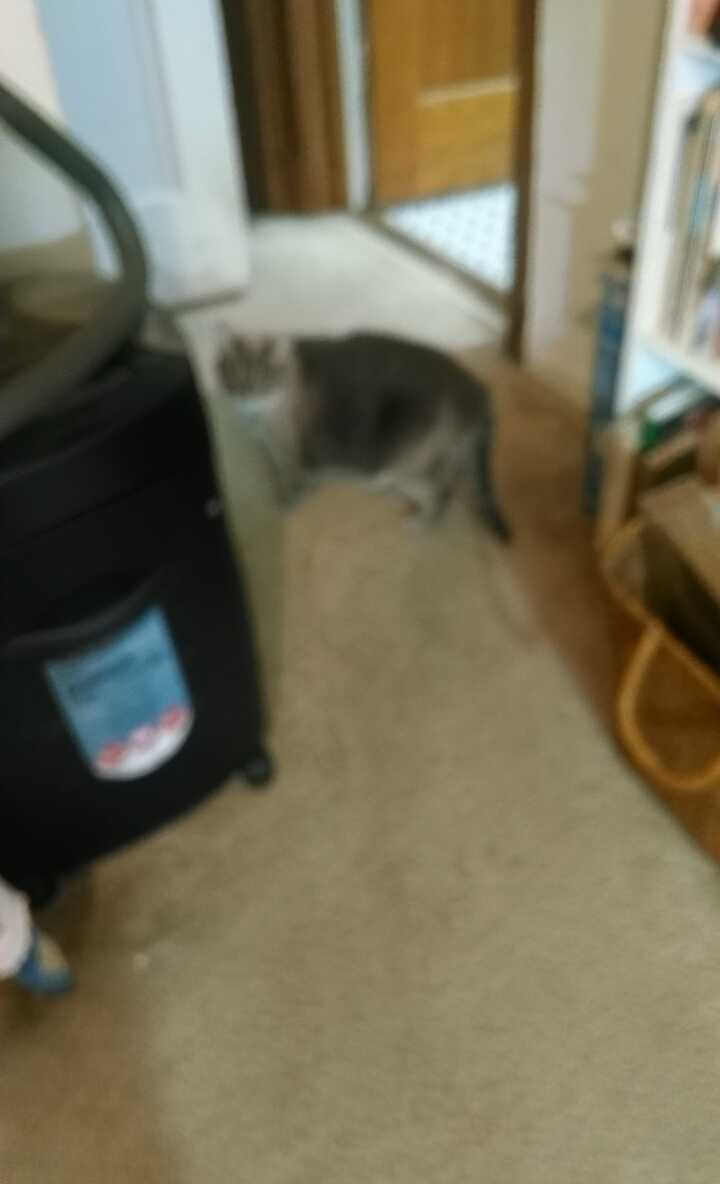This is an extremely blurry indoor photograph featuring a large grey and light grey cat standing on what appears to be beige or creamish-colored carpet. The cat, looking towards the camera, stands in the center of the image, though its features are not clear due to the motion blur. To the left of the cat is a black canister vacuum cleaner, possibly with a blue logo on it. On the right side, there's a white bookshelf filled with books, with a handle emerging from a bag or basket on the bottom shelf. In the background, there's an open timber door leading into a well-lit room with a white floor adorned with small black marks.